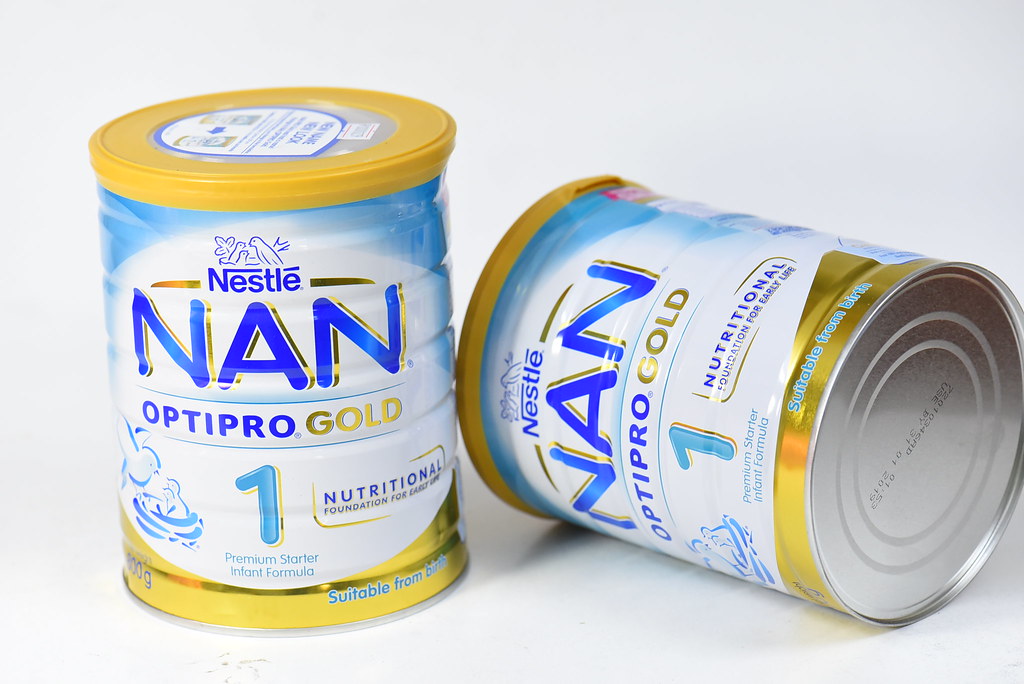This is a professional photograph of two cans from Nestlé, displaying the Nan Optipro Gold Premium Starter Infant Formula. The cans predominantly feature blue and white colors with gold accents and have a silver bottom. The can caps are yellow. The can on the left is upright, while the one on the right lies on its side. Each can displays the Nestlé logo in blue at the top, below which "NAN" is written in blue text with a golden drop shadow. Underneath, "OptiPro Gold" and the number 1 are prominently featured. Below this, the text "Premium Starter Infant Formula" and "Nutritional Foundation for Early Life" is printed. The cans are labeled "Suitable from Birth" on a gold background on the bottom right and state a weight of 100 grams in blue text on the bottom left. Additionally, there is an image of a nest with two baby birds and a mama bird flying above them. The photograph showcases the cans on a white backdrop, reminiscent of a professional studio setting. Noticeable is an expiration date of January 31, 2019, printed on the silver bottom of the cans.